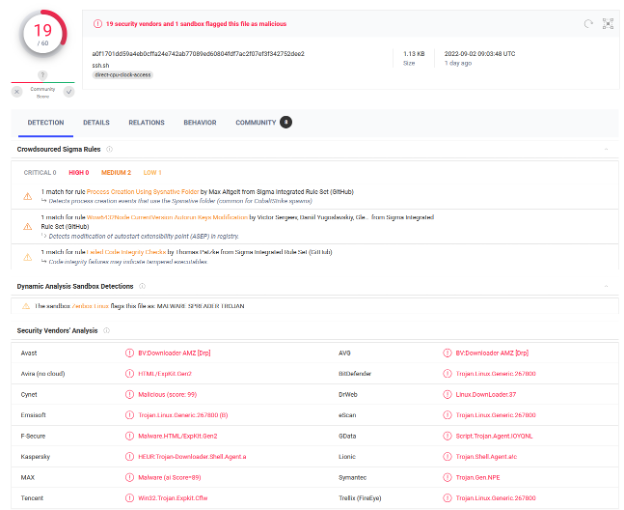The image appears to be a detailed report from a cybersecurity platform, possibly a malware detection dashboard. Here is a detailed descriptive caption for the image:

---

The left-hand side of the image features a circular graphic. The circle's outline is primarily gray but transitions to hot pink. Within the circle, the interior is white, displaying the text "19/16" in hot pink and gray respectively. Adjacent to the circle, in hot pink text, it states "19 security vendors and one sandbox flag." Below this, in black text, it reads "This file has malicious," though the text is somewhat blurry and hard to decipher. Further right, the image lists "1.13 KB" or "1.19 KB"—the exact value is unclear. Additionally, there is a date formatted as "2022-09-02" and a timestamp indicating the data is "one day ago."

The upper right of the image includes a horizontal blue navigation bar with tabs labeled "detection" (highlighted in blue), "details," "relations," "behavior," and "community." Below this navigation bar, the background turns white. In black text, it reads "crowdserved Sigma rules." There are also severity levels listed: "critical" in gray with a value of zero, "high" in pink with a value of zero, "medium" in orange with a value of two, and "low" in light orange with a value of one. The bottom section contains more black text, though it is blurry and difficult to read.

---

This caption provides a comprehensive description of all observed elements, helping users visualize the detailed report without needing to see the image itself.